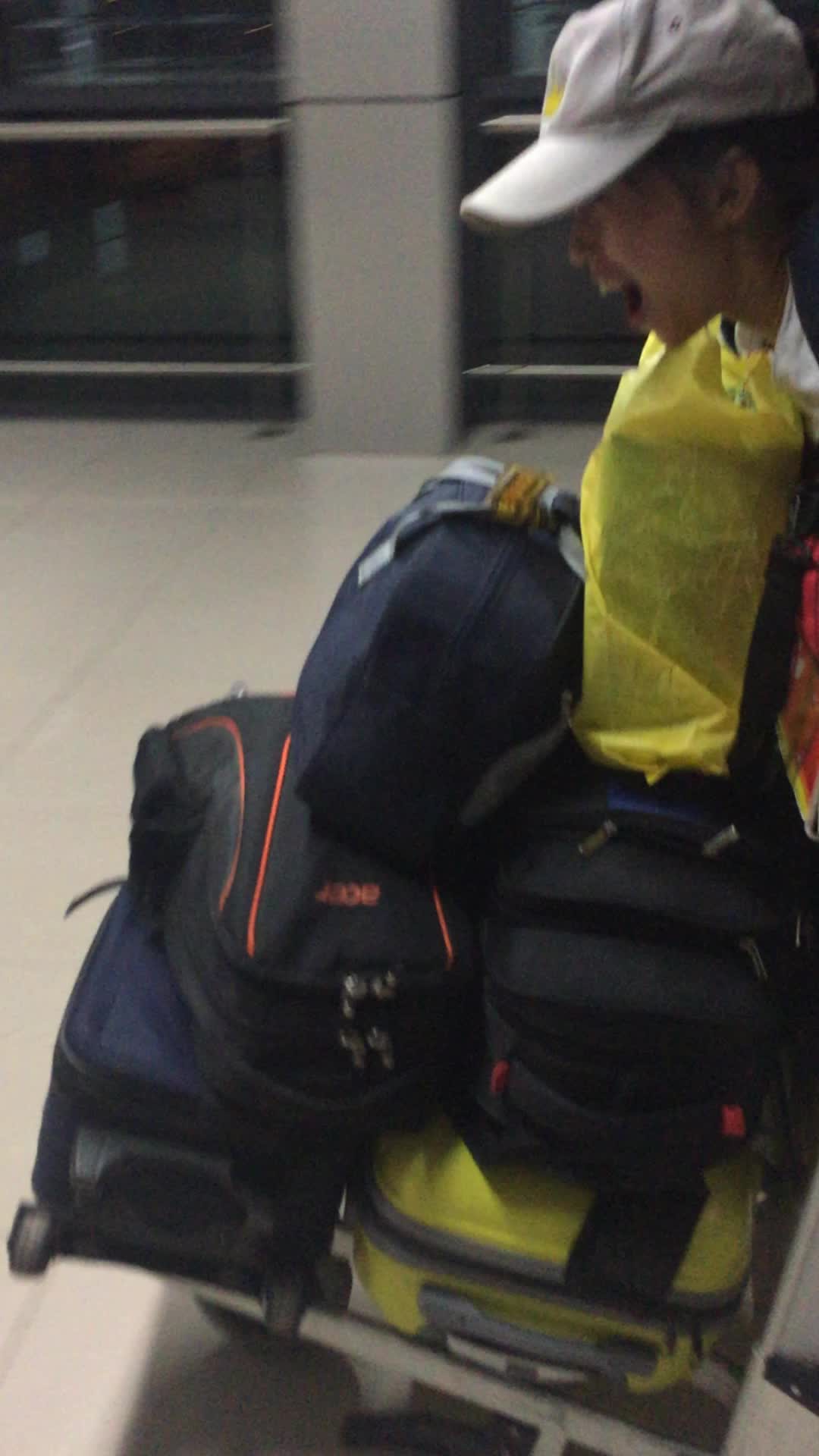In this image, we see a person whose head is visible while the rest of their body is cropped out. They are wearing a hat—either white with a yellow design or tan—with their mouth open, possibly yelling or expressing joy. The person has black hair and appears to be an airport worker, or at least someone handling luggage.

The person is managing a luggage carrier, a rolling device loaded with several pieces of luggage. At the bottom of the stack is a yellow suitcase, and next to it on the left is a navy blue suitcase. On top of the navy blue suitcase is a black bag with red striping, while on top of the yellow suitcase is a plain black bag. Above these is another navy blue bag, possibly a bathroom bag, and at the very top sits a yellow store bag. This metal luggage carrier is on a white linoleum floor, and it looks heavily loaded, capturing a moment of bustling activity.